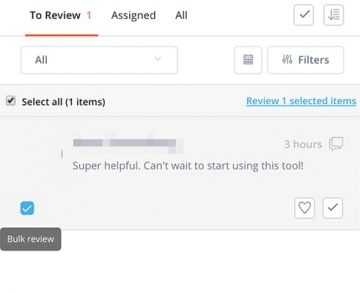The image appears to be a cropped screenshot of an unidentified application or website interface, likely a dashboard for managing tasks or reviews. 

In the top left corner, the interface features a white background with black text reading "To Review," accompanied by a red number "1" indicating the count of items pending review. To the right, there are two additional tabs labeled "Assign" and "All." The "To Review" tab is highlighted with a red underline, indicating the current active category.

In the upper right corner, there is a black checkmark icon outlined in black, next to what seems to be a drop-down menu icon.

Below the main navigation tabs, there is a pull-down box labeled "All," followed by icons that likely represent a calendar link and a filters link, allowing further sorting and selection options.

In the main content area under the "To Review" section, there is an option to "Select All Items," which applies to one item, and it has been checked. To the right of this, in blue font, there is a link labeled "Review 1 selected item."

Beneath this section, the message under review reads: "Super helpful. Can't wait to start using this tool!"